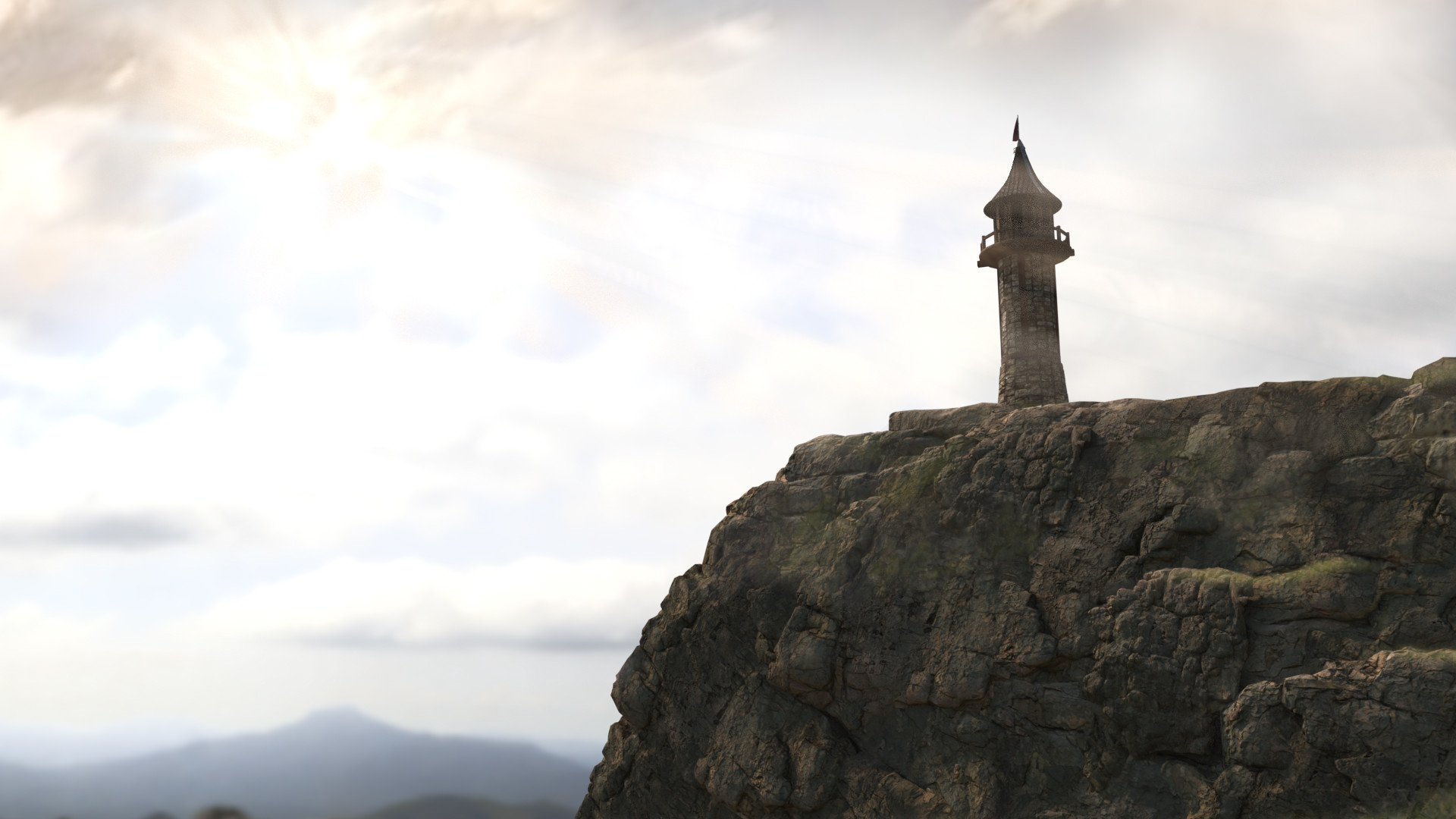A rectangular image, oriented horizontally, showcases a dramatic scene that blurs the lines between photography and digital artistry. At the center of this composition stands a large rocky outcrop, deeply textured in shades of dark gray. Perched atop this rugged formation is a tower, reminiscent of a lighthouse, possibly adorned with a flag fluttering at its peak. The distant background reveals a range of mountains nestled in the bottom left corner, adding depth to the scene. Dominating the rest of the image, a vast, cloudy sky stretches across, painted in varying hues of blue. From the upper left, the sun breaks through the cloud cover, its rays casting a celestial spotlight on the tower and rock, enhancing the mystique and grandeur of the landscape.